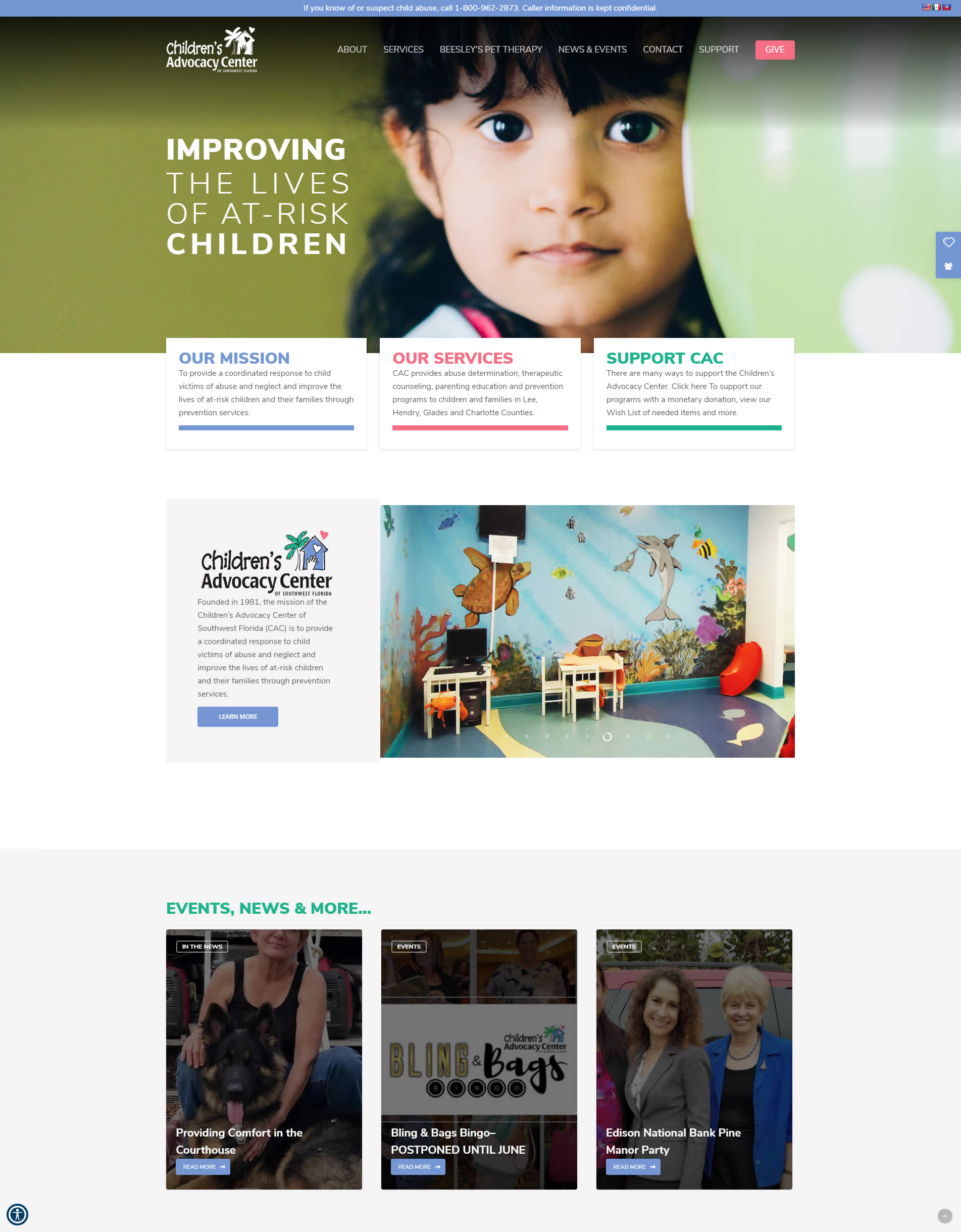The website of the Children's Advocacy Center prominently features a large, detailed header. At the very top, a thin blue border contains a vital phone number for reporting or inquiring about child abuse. Below this, the header transitions into a green background showcasing the face of a young girl with black hair and caramel-colored skin. Adjacent to her on the left, the text reads, "Improving the lives of at-risk children."

Beneath the main header, three distinct white square tiles are presented. The first tile, accented with blue at the top, is labeled "Our Mission." The second tile, highlighted in red, is labeled "Our Services," while the third tile, in green, invites viewers to "Support CAC" (Children's Advocacy Center).

Further down, a larger white block on the left side of the page prominently displays the name "Children's Advocacy Center," accompanied by information about their services and programs.

To the right of this information block, there's an image of a room featuring a vibrant mural of an aquarium, with tables, chairs, and an aquatic-themed decor extending to the floor.

At the bottom of the page, the section titled "Events, News, and More" showcases three separate tiles, each detailing different events hosted by the Children's Advocacy Center.